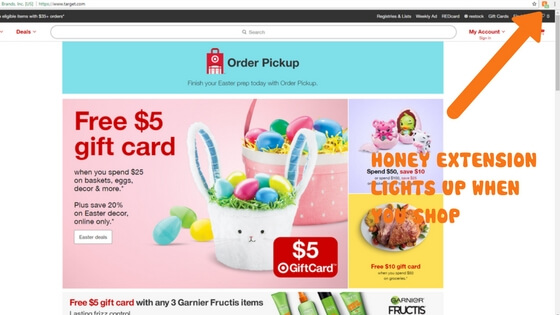Screenshot of a desktop computer displaying product documentation for the Honey browser extension. A large, diagonally placed orange arrow points to the top right corner of the screen, where a small Honey icon is visible. Below the arrow, bold capitalized text reads, "HONEY EXTENSION LIGHTS UP WHEN YOU SHOP," indicating the visibility status of the Honey extension. Next to the Honey icon, there's a green notification likely informing the user about potential savings.

The main content on the screen is a Target order pickup page, featuring an Easter-themed flyer. The flyer prominently displays an Easter Bunny basket holding colorful Easter eggs with a note saying "FREE $5 GIFT CARD" in red text against a pink background. Above the flyer, there is a light blue banner labelling the page as "Order Pickup," accompanied by the Target logo in red on the left.

If the user were to scroll up, they would see an advertisement for Garnier Fructis. The ad mentions a deal: "FREE $5 GIFT CARD with any three Garnier Fructis items," with green Garnier Fructis product bottles partially visible at the bottom of the screenshot.